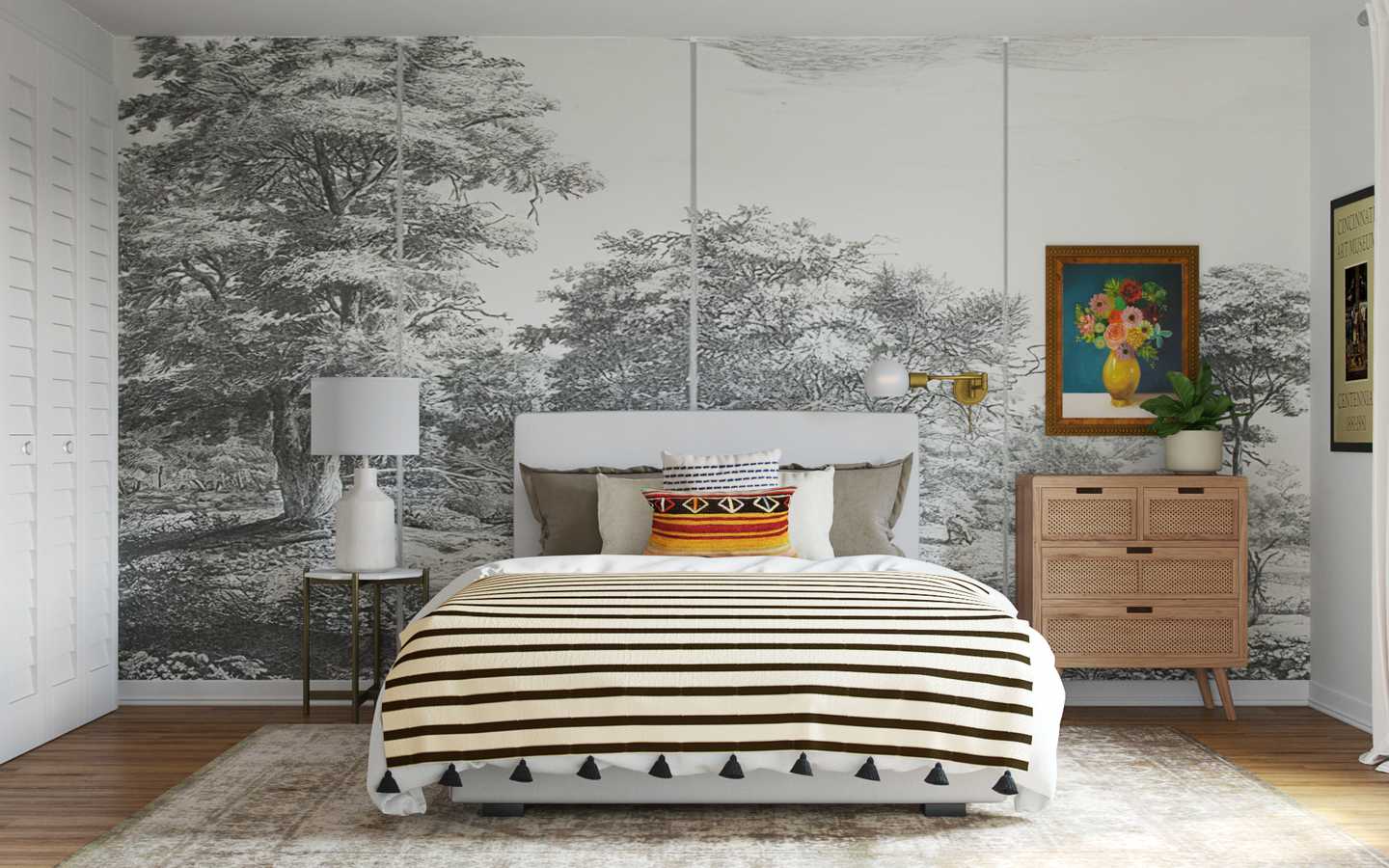The image captures the interior of a modern, well-organized bedroom bathed in natural daylight. Dominating the room, at the center, is a white bed with a white backboard. The bed is adorned with various pillows, including beige and white ones, accompanied by a striking yellow, red, black, and white pillow in the middle. A beige blanket with black stripes and triangular fringe drapes over the white bedsheet. The scene is not merely confined to the bed; a large, bright rug sits beneath it, anchoring the room's design.

On the wall behind the bed, there's a stunning black-and-white mural depicting a serene garden or meadow, complete with a large tree on the left, smaller trees in the middle, and another smaller tree on the right. This mural is divided into four distinct panels, creating a striking visual focal point. To the left, white closet doors add to the room's modern feel, while on the right, there's a wooden dresser topped with a painting of colorful flowers. Directly above the dresser, a credenza holds another small floral painting. By the bed, an end table supports a sleek white lamp.

The room's wooden floor adds warmth to the décor, contrasted by a large area rug under the bed. The entire space is meticulously organized, capturing a clean, aesthetically pleasing, and beautifully designed sanctuary.